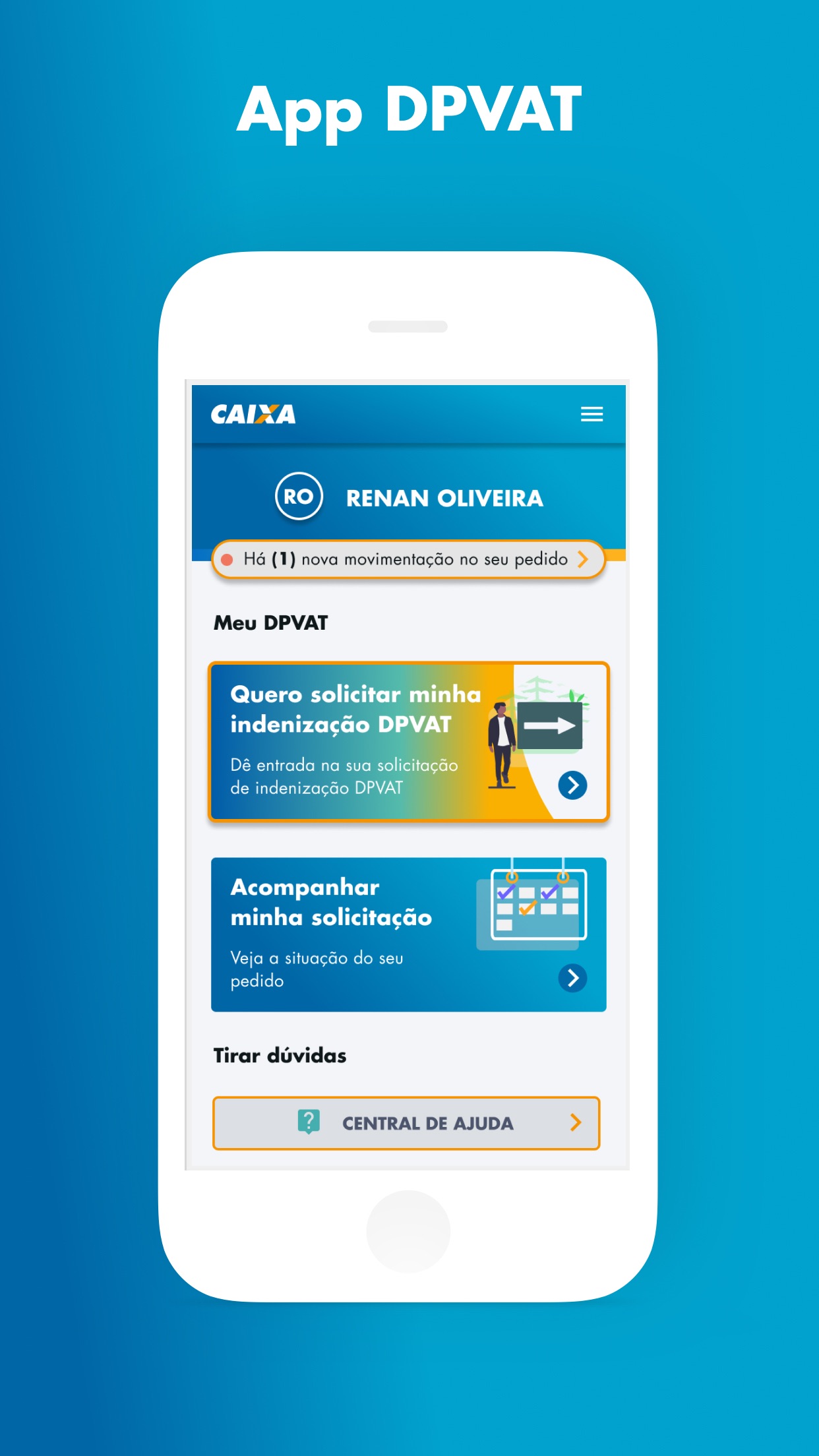This illustration showcases a smartphone app advertisement set against a blue background in portrait orientation. At the top, in white text, the app is identified as "App DPVAT." The app interface is displayed on a neutral white phone with the company logo "CAIXA" in capital letters on the upper left and a hamburger menu on the upper right. 

Below the header, the name "Renan Oliveira" is prominently featured, accompanied by the initials "R.O." inside a blue circle with a white border. A notification marker "HA1" can be seen, and the text on the app is primarily in a non-English language. The phrase "MEU DPVAT" is visible next, indicating a potential section or feature of the app.

Further down, there are graphical blocks and various text elements: one block includes an icon of a person walking along with an arrow; another block features a calendar icon redirecting to another section. At the bottom, the text "Central de Ajuda" (which translates to "Help Center") is displayed, providing users with an option for assistance.

This detailed illustration highlights various elements of the app, focusing on its layout and features, despite the language barrier.